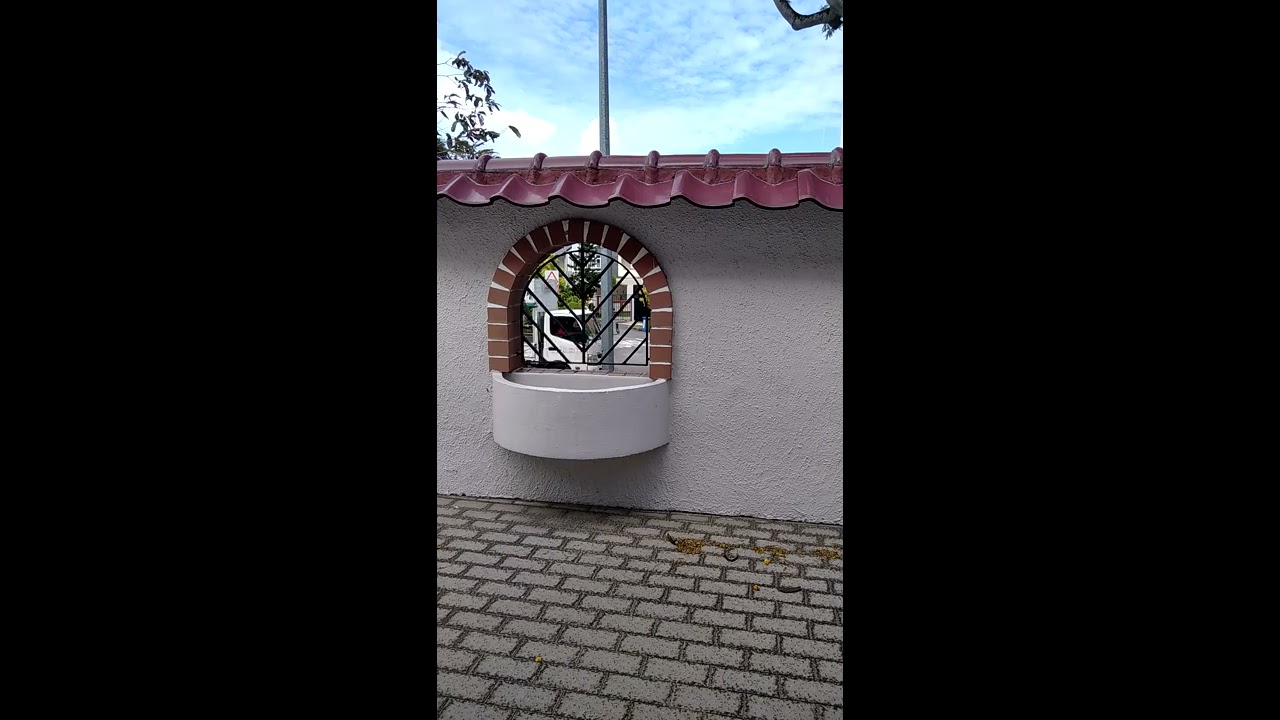This detailed photograph features the side of a building with distinct architectural and natural elements. The central focus is a gray, cement wall with a rough textured surface, spanning the width of the vertically oriented image. In the middle of the wall, there is an arched opening framed by a row of red bricks held together with white mortar. Inside this arch is an intricate metal gate composed of black bars, with one bar extending straight down and others branching diagonally to the left and right.

Directly below the arched window is a round, concrete catch, likely a planter or water collector. The ground in front of the wall is paved with gray bricks set in darker gray mortar. Above the arch, the building features a maroon-colored metal roof with a scalloped, wavy design, extending slightly over the edge of the wall. Through the arch and at the top of the structure, a silver metal bar is visible, rising vertically.

Surrounding this central structure, hints of nature appear in the form of leaves and branches on the left side and upper right corner of the image. The sky in the background is painted in light shades of white and blue with soft clouds, contributing to the serene environment captured in this scene.